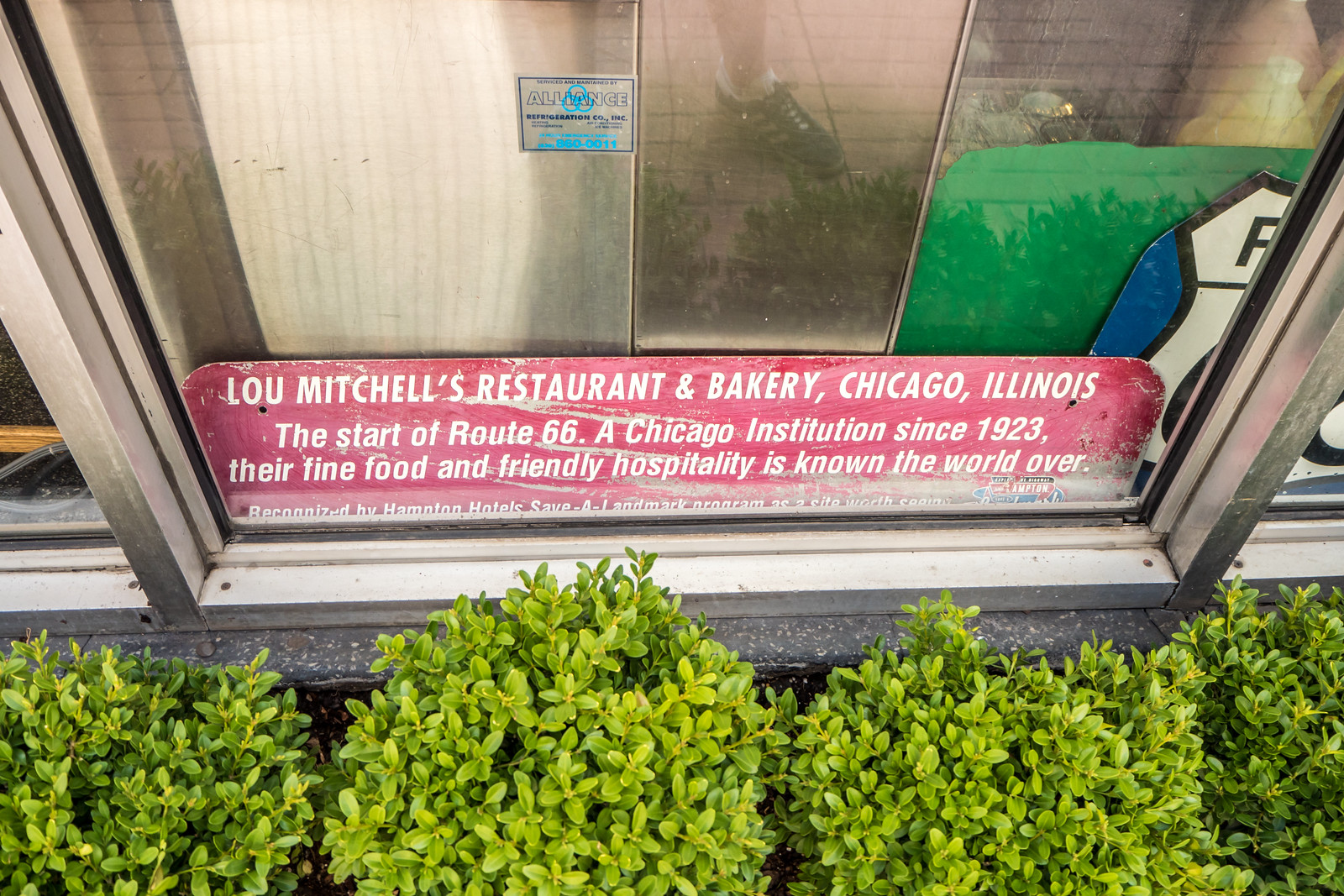The photograph showcases the storefront of Lou Mitchell's Restaurant and Bakery, located in Chicago, Illinois. The very forefront features four meticulously manicured small green bushes. Above them is a silver-framed single-pane window, which makes up the storefront. Dominating the window is a red rectangular sign with curved edges and white font that reads: "Lou Mitchell's Restaurant and Bakery, Chicago, Illinois. The start of Route 66, a Chicago institution since 1923. Their fine food and friendly hospitality is known the world over, recognized by Hampton Hotel's Save a Landmark program as a site worth seeing." Inside the window, towards the right side, there is a partially obscured Route 66 road sign. Additional items, including something green, a white shade, and a blue and white sign with the letter 'F' also appear inside the window, contributing to visual blocking. Reflections on the glass show what appears to be the photographer's foot, clad in white socks and black and gray tennis shoes, hinting at an exterior daytime scene.